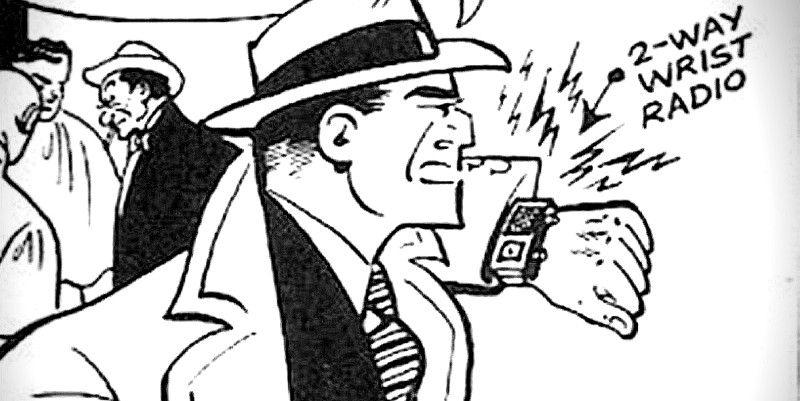The black and white panel from an old Dick Tracy cartoon, likely from the 50s or 60s, features Dick Tracy in profile, facing right. He dons a distinctive white trench coat with the collar pulled up, a dark suit, a white and black striped tie, and a white fedora with a black band. With a fierce expression, Tracy holds up his left arm, speaking into or listening to his iconic two-way wrist radio, indicated by sound wave symbols and labeled as such. Behind him, three men huddle in conversation; one wears a black jacket and has a cigarette, another a black coat and white hat with a bulbous nose, and the last two, wearing white shirts, might be doctors. The scene is animated with energy lines emanating from the radio, emphasizing Tracy's urgent communication.